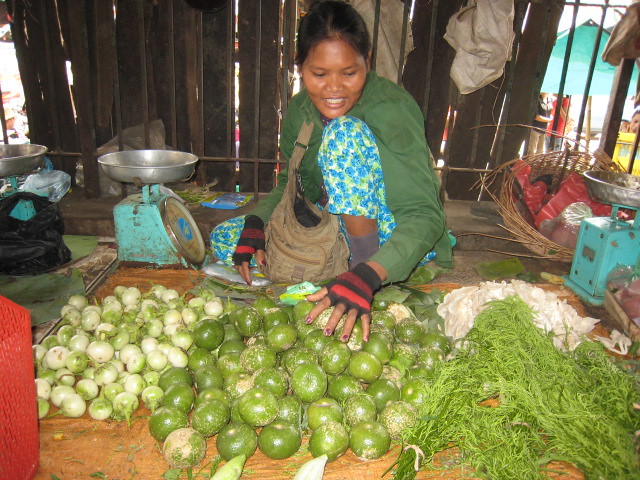In the image, an Asian woman with dark skin and brown hair is kneeling at a vegetable market stall. She is wearing a green shirt and vibrant blue pants adorned with floral patterns, along with red and black fingerless gloves that reveal her purple nail polish. A brown sling bag is draped across her chest. Surrounding her are various fruits and vegetables, including lime-like fruits, white and green onions, and leafy, stringy vegetables. Metal bowls and several old, rusty scales with stainless steel cups are also present, indicating she is likely weighing produce. The market setting features a wooden raised platform covered with carpets and cloths, additional plastic and paper bags, and baskets. Behind her, a wall made of wooden planks separates her from the bustling market where more people are visible. A canopy overhead suggests the market is outdoors and the sunlight indicates that the photo was taken during the daytime.